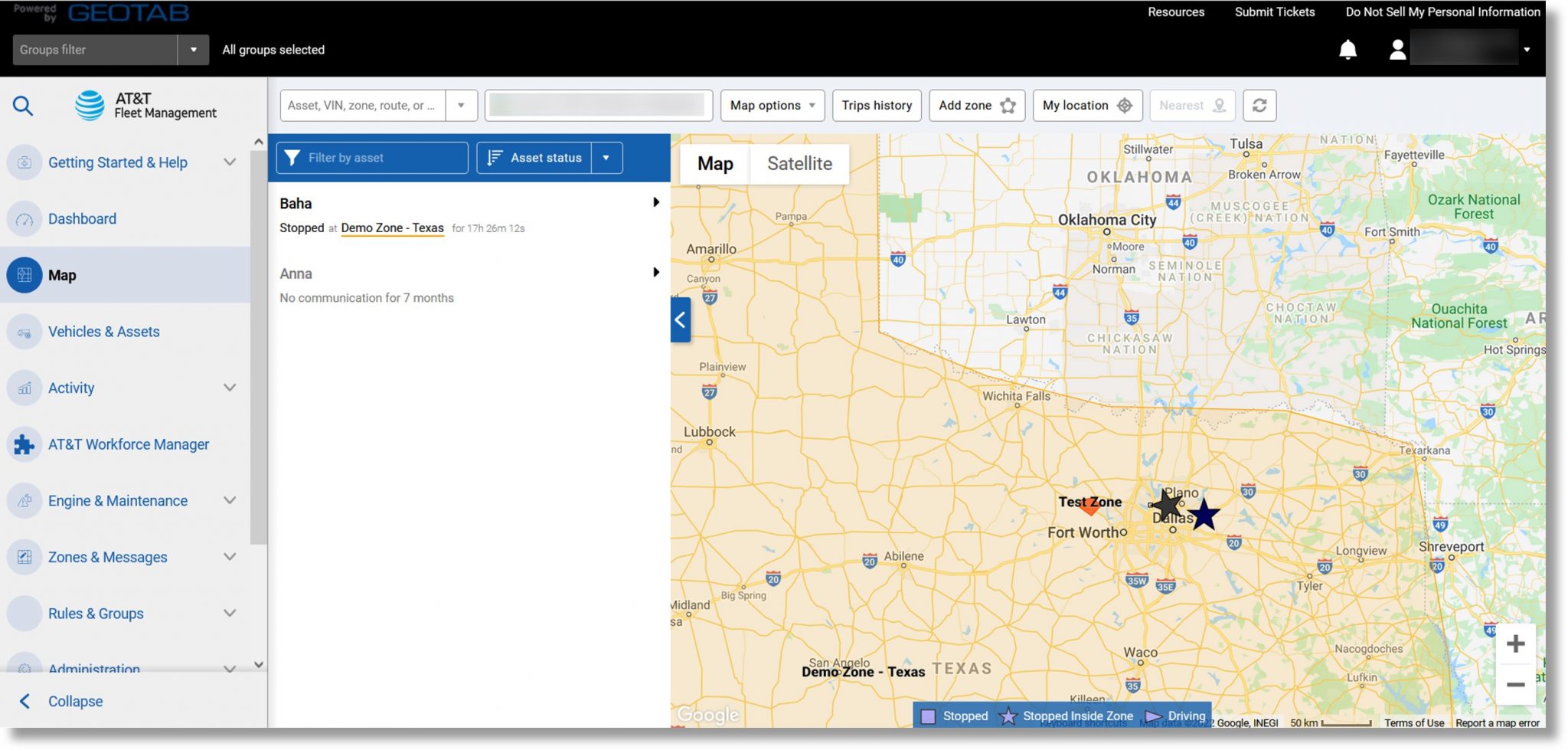Cropped screenshot of the GeoTab website.

At the top, a black header spans the width of the page, displaying the "GeoTab" logo in the top left corner. Directly beneath this, a gray drop-down box is located on the bottom left.

On the right side of the header, three small white-text categories are neatly aligned: "Required," "Submit Tickets," and "Do Not Sell My Personal Information." Below these categories, to the bottom right, a bell icon and an account icon are visible, with the account information pixelated for privacy.

Moving to the main body of the page, the top left corner features the "AT&T Fleet Management" logo. Beneath this logo is a vertically arranged menu of categories, with the "Map" category currently selected.

To the left of the main content area, a white panel houses a "Filter by Asset" box, next to which is a drop-down set to "Asset Status." Below this filter section, the panel lists two vehicles. The first vehicle, named "Baja," is marked as stopped at a specific location. The second vehicle is indicated by a grayed-out icon, suggesting it is not in service.

Dominating the right side of the page is a large map extending to the far edge, featuring two stars that denote the locations of the two vehicles mentioned.